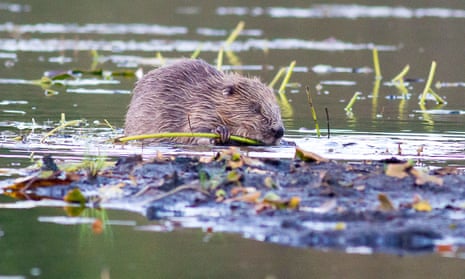The photograph captures a beaver in murky green water, with numerous green stems and plants protruding from the surface. The close-up perspective reveals the beaver holding onto a partially eaten stem, its eyes closed as if taking a nap. The water appears green and reflective, with muck visible in the lower part of the image beneath the beaver. The top of the photo blurs into more water, adding to the serene yet industrious scene. The beaver seems to be preparing materials, possibly to build a dam, deepening the natural, tranquil atmosphere of the moment.